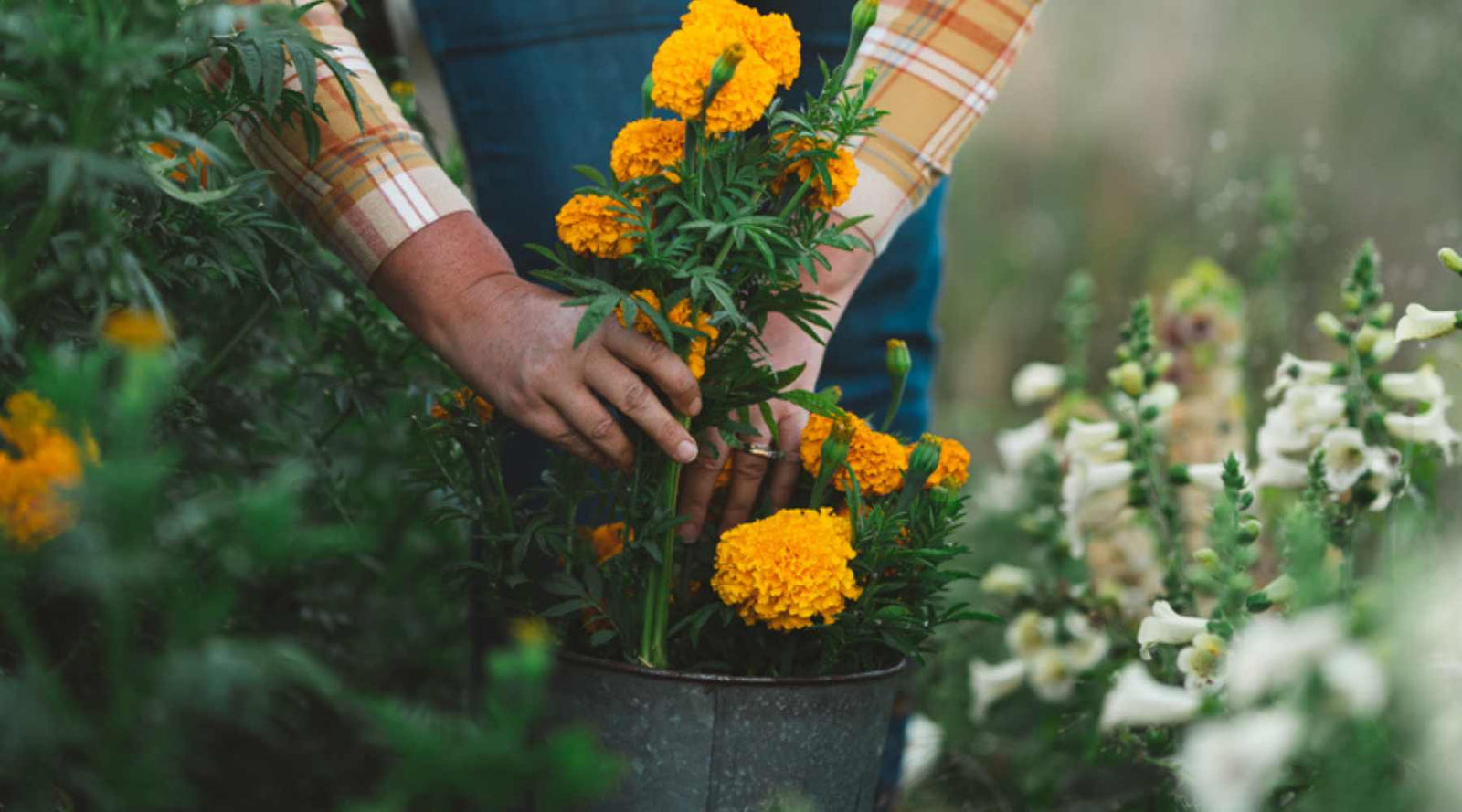Amidst a vibrant garden, the focus of the image rests on the hands of a gardener, partially visible and clad in blue jeans, a long-sleeved plaid shirt in hues of orange, yellow, and white, and a blue apron. The gardener is carefully placing bright orange-gold flowers, resembling marigolds, into a slightly rusted, galvanized metal pail. Surrounding the gardener are lush green plants, with stocky stems of sweet peas on the right side and foxglove flowers appearing further back. The image is artfully blurred at the edges, drawing attention to the detailed work of the gardener's hands in the center, embodying a moment of serene dedication amidst a sea of flora.